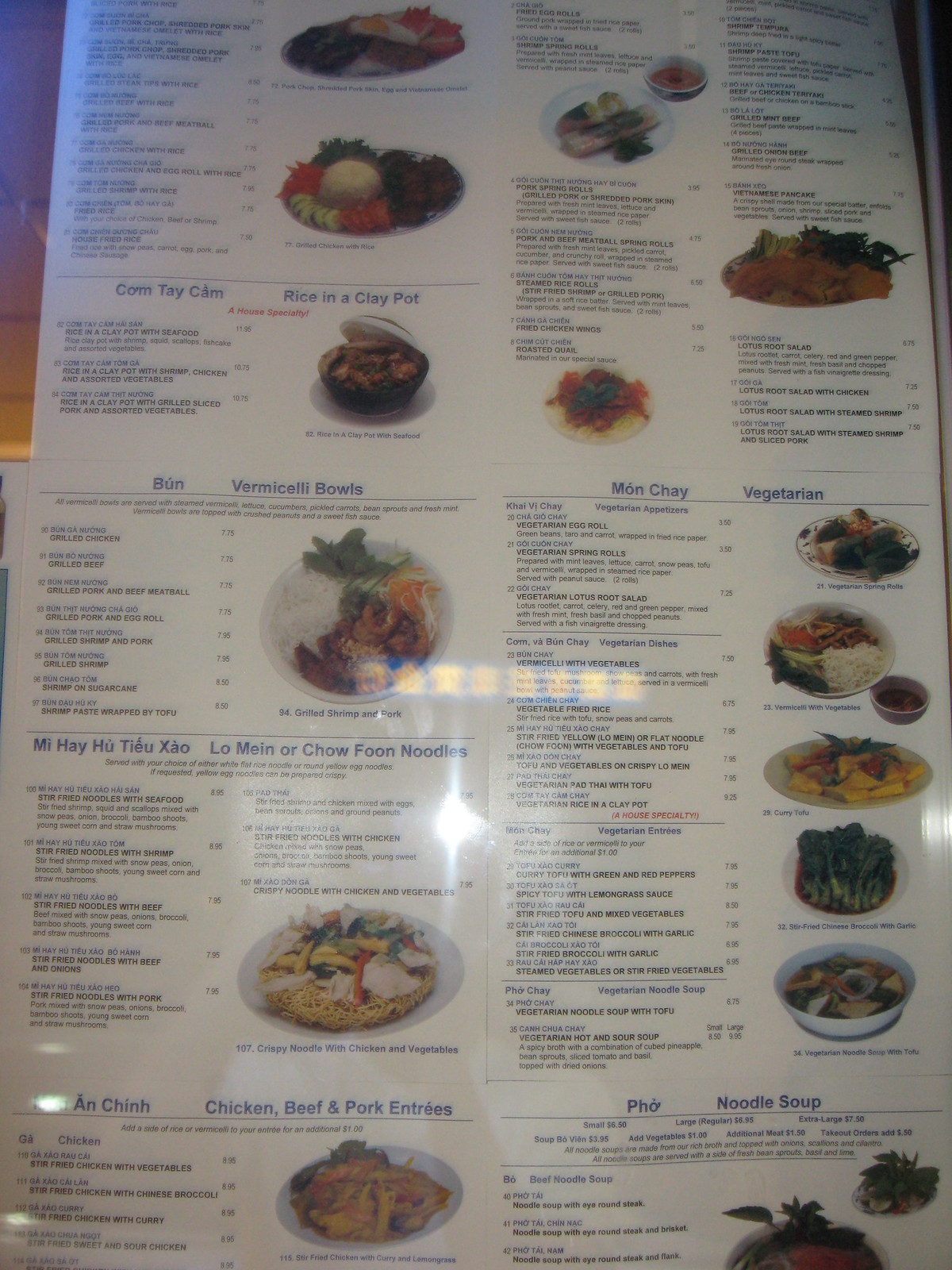Close-up image of a partially visible menu with an oriental theme. The top left corner reveals a bit of a wooden table or counter. The menu fills the entire frame, showcasing an array of dishes with diminutive text that's difficult to read. 

On the top section, a small section displays the words "come, take, cam," followed by a black-and-white image of a bowl labeled "Rice and Clay Pot" filled with food. Just above this, there’s a large oval plate with rice, surrounded by vegetables and meat. There’s another plate above this oval one. 

In the upper right section, there's a bowl with food and a plate next to it, though the writing is illegible. The bottom of the image features a white plate with red, green, and brown food items. To the far right, a large platter with a mix of greens, meat, and vegetables is visible. 

In the middle area, the word "B-U-N" appears, introducing the "Vermicelli Bowls" section, accompanied by a big white bowl filled with broccoli, orange items (possibly shrimp), meat, and rice. Below this, there’s a section that says "lo mein" or "chow food, noodles," followed by more text and an image of a white plate with noodles, vegetables, and white rice. 

The "Chicken, Beef, and Pork Entrees" section features a dish titled "An Chin" (uncertain pronunciation) showcasing vegetables and possibly chicken. In the far upper middle, the "Vegetarian" section presents a plate of green and white vegetables. Accompanying the text is a bowl with white rice and possibly a dipping sauce or soup. 

There's also a large white platter with a variety of foods, including a brown gravy-like bowl and likely broccoli. Additionally, a white bowl contains a mix of aliments. The right bottom section labeled "Noodle Soup" shows part of a big bowl with green leaves and soup, and another partially visible dish behind it.